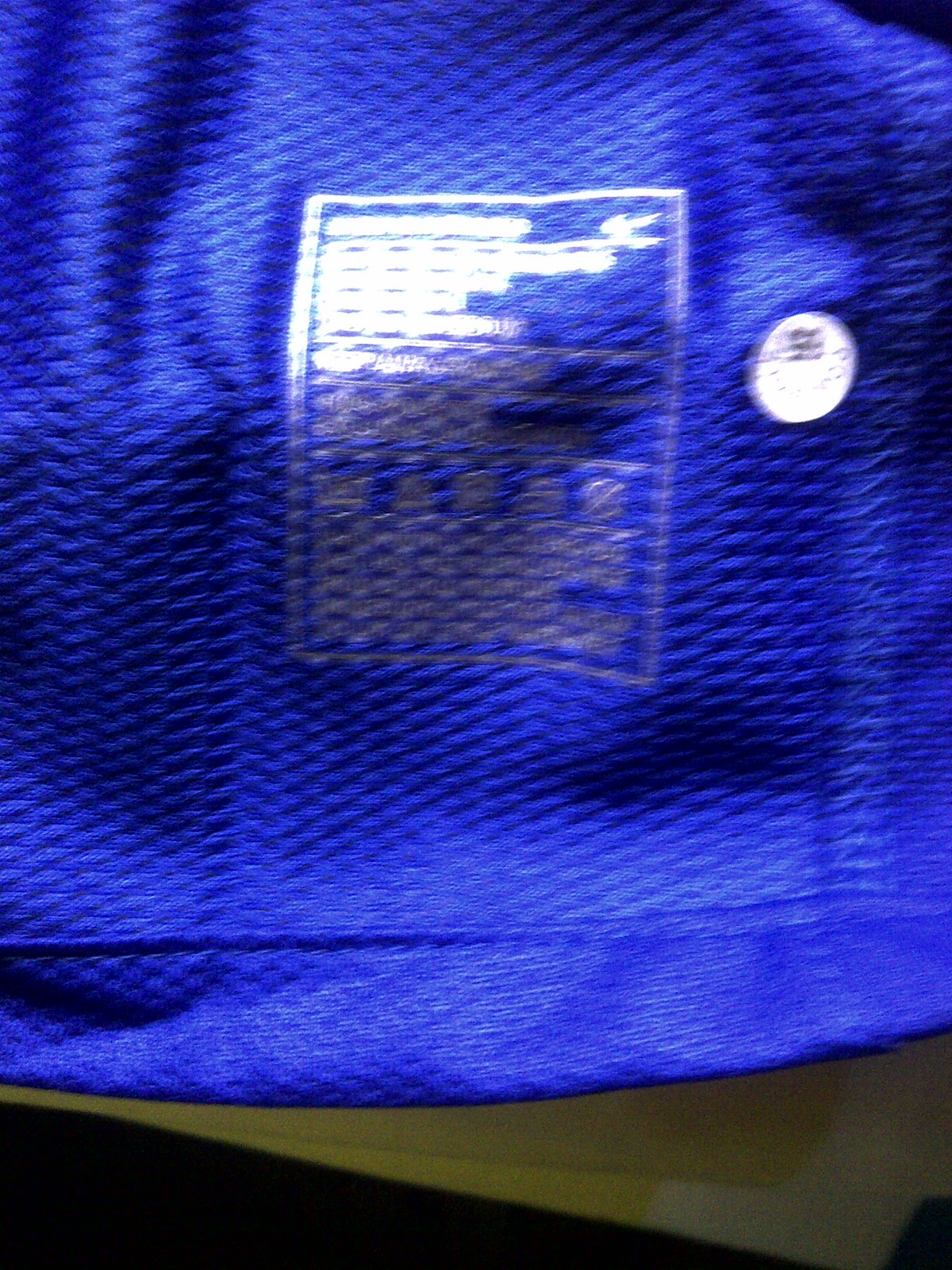This is a close-up photograph of a very textured, vivid royal blue fabric, reminiscent of that used in athletic clothing such as football jerseys. The bright blue material, which dominates most of the image, features a ridged square pattern. In the center, there is a slightly blurred silver label with some abstract design or writing that is difficult to decipher. To the right of the label, a white circular disc with undecipherable details appears, perhaps a button. The bottom fourth of the image reveals a black and gray surface, likely a table, contrasting with the vibrant blue fabric above.